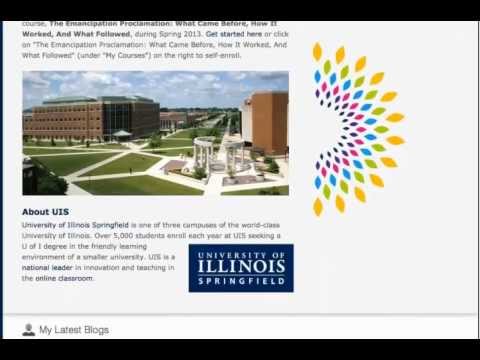This image is a screenshot of a website, though the specific site is not identifiable. The screenshot has two black bars at the top and bottom. The background of the webpage is predominantly white. Central to the image is a blue rectangular box with text in white reading "University of Illinois Springfield." Adjacent to this text box is an abstract design featuring black, pink, blue, green, and orange colors.

The focal point of the image is a photograph of a couple of buildings. The building on the left appears to be about four stories high with a brown exterior. The building on the right is slightly taller and also brown, with what seems to be a white building set behind it. Bright white walking paths crisscross between the buildings. In the foreground of the image, there are green bushes and a tree located in the left corner. The sky above is blue with scattered clouds. The clarity of the photo is somewhat compromised, resulting in a blurry appearance. At the bottom of the screen, text reads "about UIS. It's the University of Illinois Springfield," followed by "my latest blog."